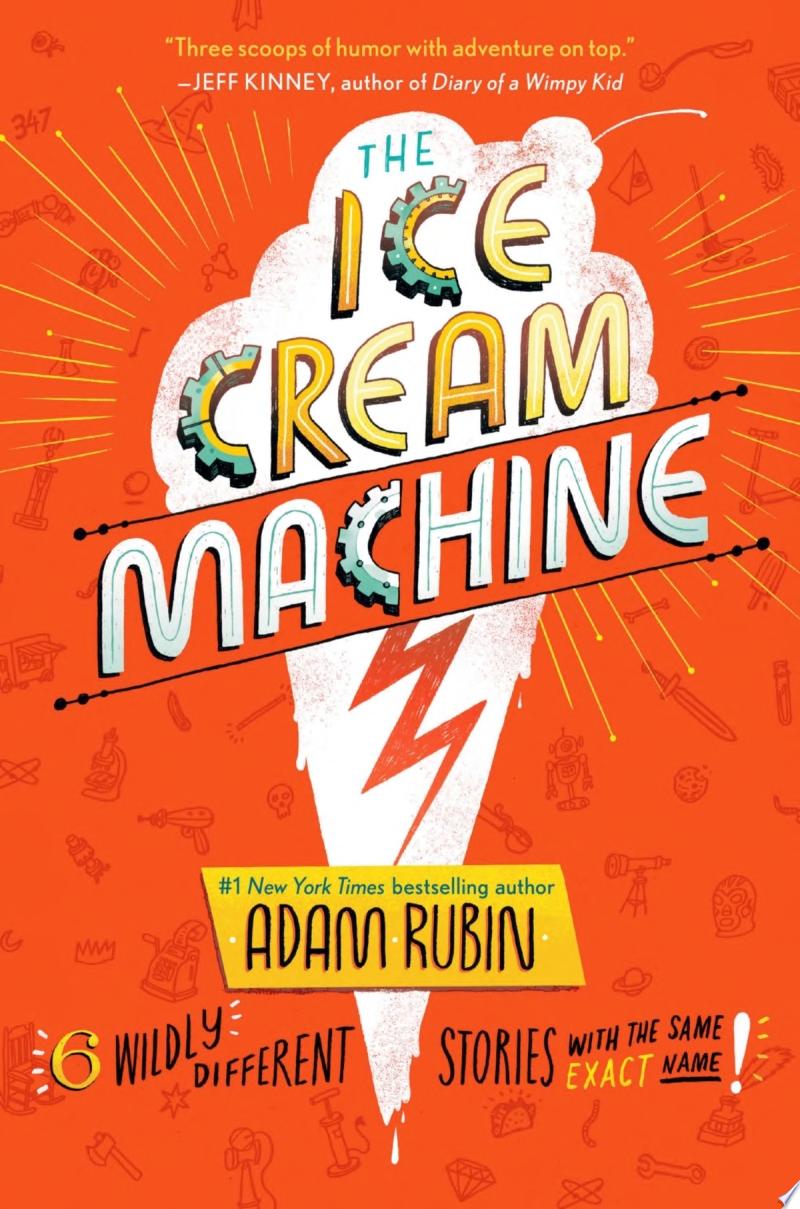This image depicts the vibrant cover of the book "The Ice Cream Machine," designed in a portrait layout where the height is shorter than the width. Dominated by a bright orange background, the cover features various semi-transparent dark orange illustrations such as a laser gun, skull, microscope, luchador mask, taco, and diamond. The lower right corner of the cover is slightly turned up, revealing a white underside.

Central to the design is a white ice cream cone with an orange lightning bolt running through it. The book’s title, "The Ice Cream Machine," is creatively placed at a slight diagonal from the bottom left to the top right, with the letters "C" in both "Ice" and "Cream" stylized to resemble cogs. Above the title, a yellow banner reads, "Three scoops of humor with adventure on top," attributed to Jeff Kinney, author of "Diary of a Wimpy Kid." Below the cone, another yellow banner states, "Number one New York Times bestselling author," followed by the author’s name, Adam Rubin. At the very bottom, a description asserts, "Six wildly different stories with the same exact name!"